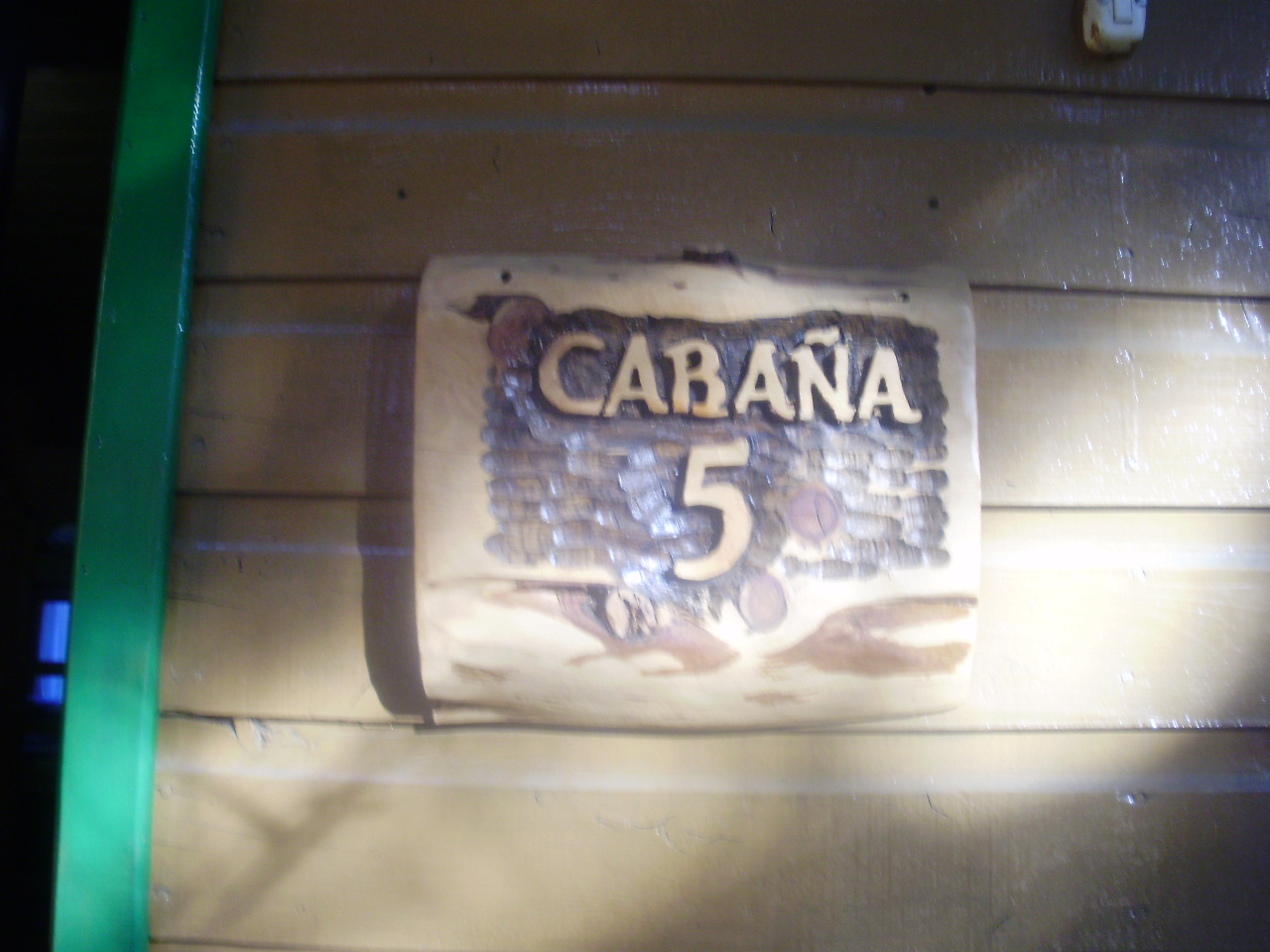The photograph captures the entrance to a rustic cabin, specifically marked as "Cabana 5" with a distinct wooden sign. The sign, crafted with intricate woodworking, features the text "Cabana 5" etched and stained to a glossy finish, complete with a tilde over the "n," indicating its Spanish origins. The sign is mounted on a brown wooden wall, with the natural grain and paneling of the wood visible beneath a layer of paint. To the left of the sign, a doorway trimmed in aqua green is partially visible, offering a slight peek into the dark interior of the cabin where a blue-lit window can be faintly seen. Additionally, a white, somewhat rusted device is affixed to the top right corner of the wall, adding to the rustic charm of the scene. The image is softly lit and somewhat out of focus, enhancing the warm, inviting ambiance of this secluded retreat.